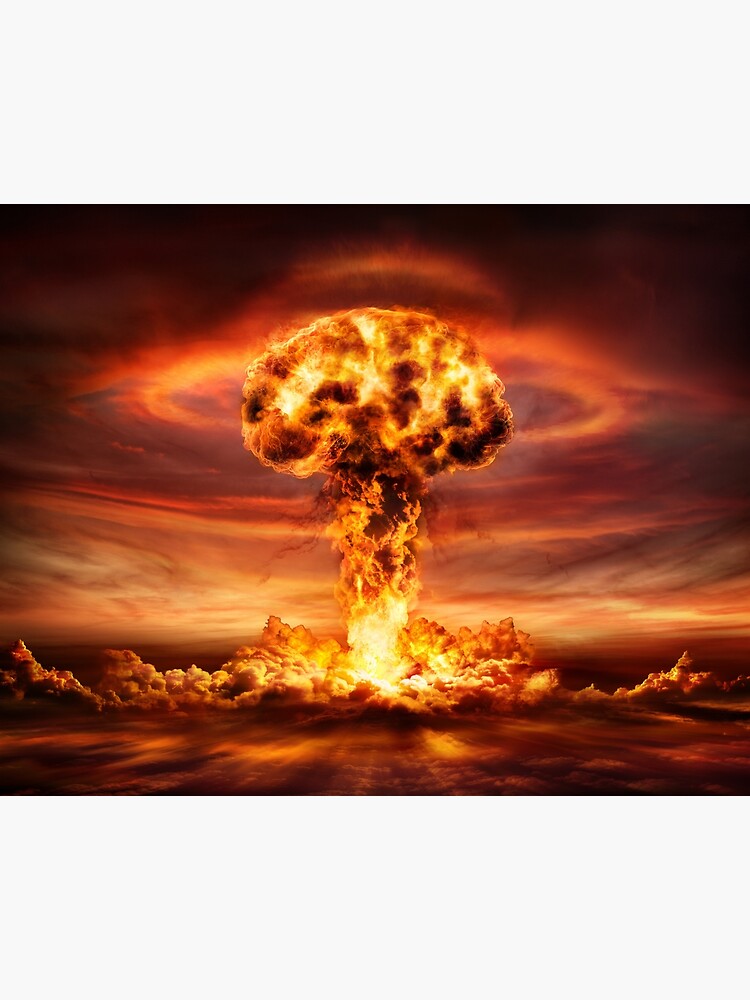The image depicts an intense, apocalyptic scene dominated by a massive, fiery mushroom cloud that appears to result from a nuclear explosion. The central plume of fire and smoke rises dramatically, illuminated by deep hues of orange, red, and yellow. Flames are visible both at the base, where the explosion originated, and within the soaring mushroom cloud, accentuating the inferno. The sky above is dark and foreboding, with black and orange clouds swirling around the plume's head, creating an almost ethereal ring of light. The landscape is minimal, suggesting a barren or desert setting, overwhelmed by the explosive spectacle. Portions of light and color extend outward from the center, evoking a sense of reverberation and dispersal of energy, with some observers noting a faint, UFO-like appearance due to the dispersion of light.